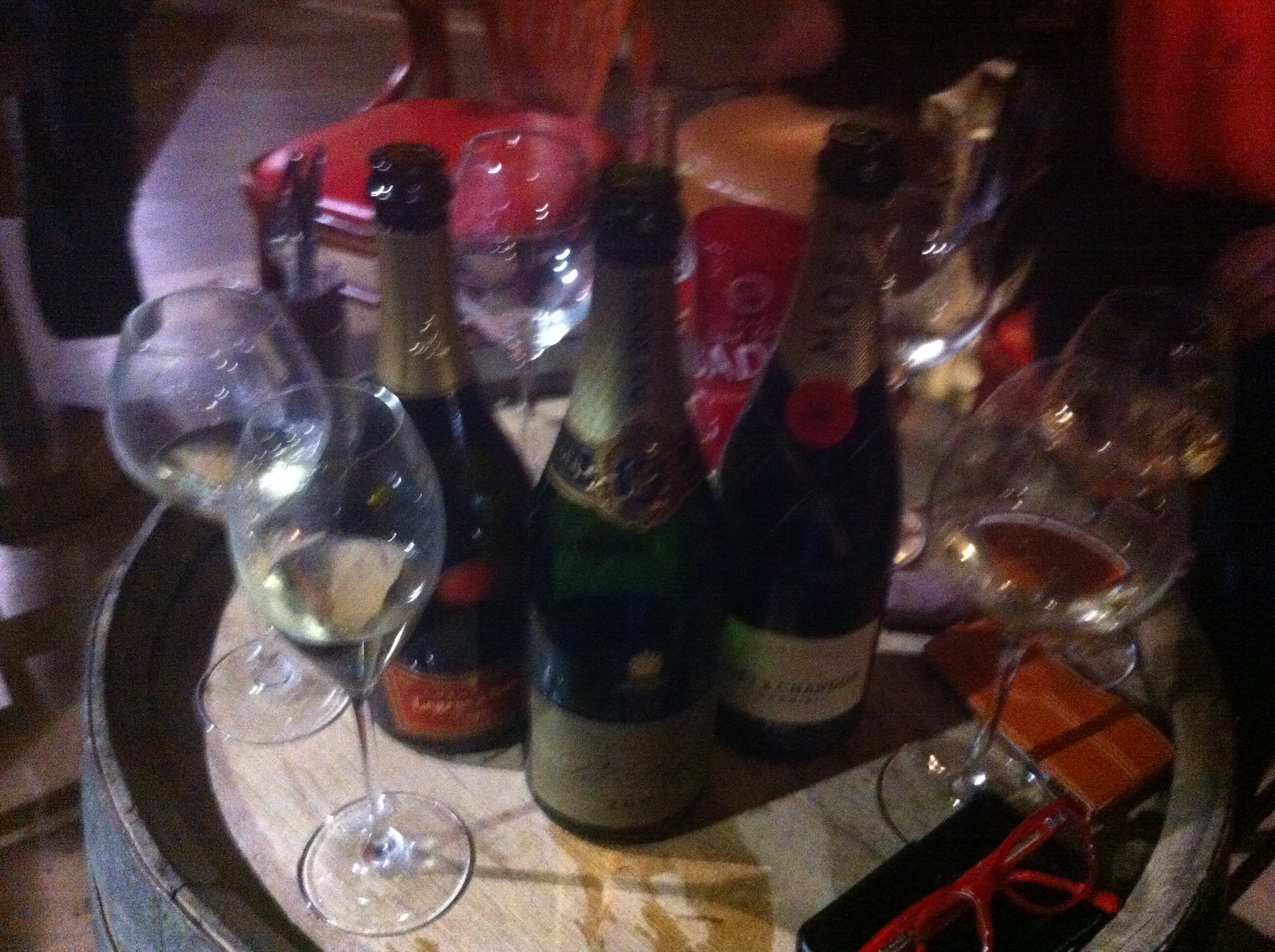The photograph portrays a dimly lit, blurry scene centered on a wooden barrel repurposed as a table. The lighting is poor, with a single light source creating a discernible glare. Atop the barrel table is an array of items: three uncorked wine bottles, one recognizable as Moet, and several wine glasses, some with partial fills of champagne and various wines. Scattered also are objects like a tan brown leather phone case with a phone and a pair of red-rimmed glasses situated near the bottom right corner. In the background, a red-cushioned wooden chair is faintly visible. The scene captures a cozy yet indistinct ambience, suggesting a bar-like setting.